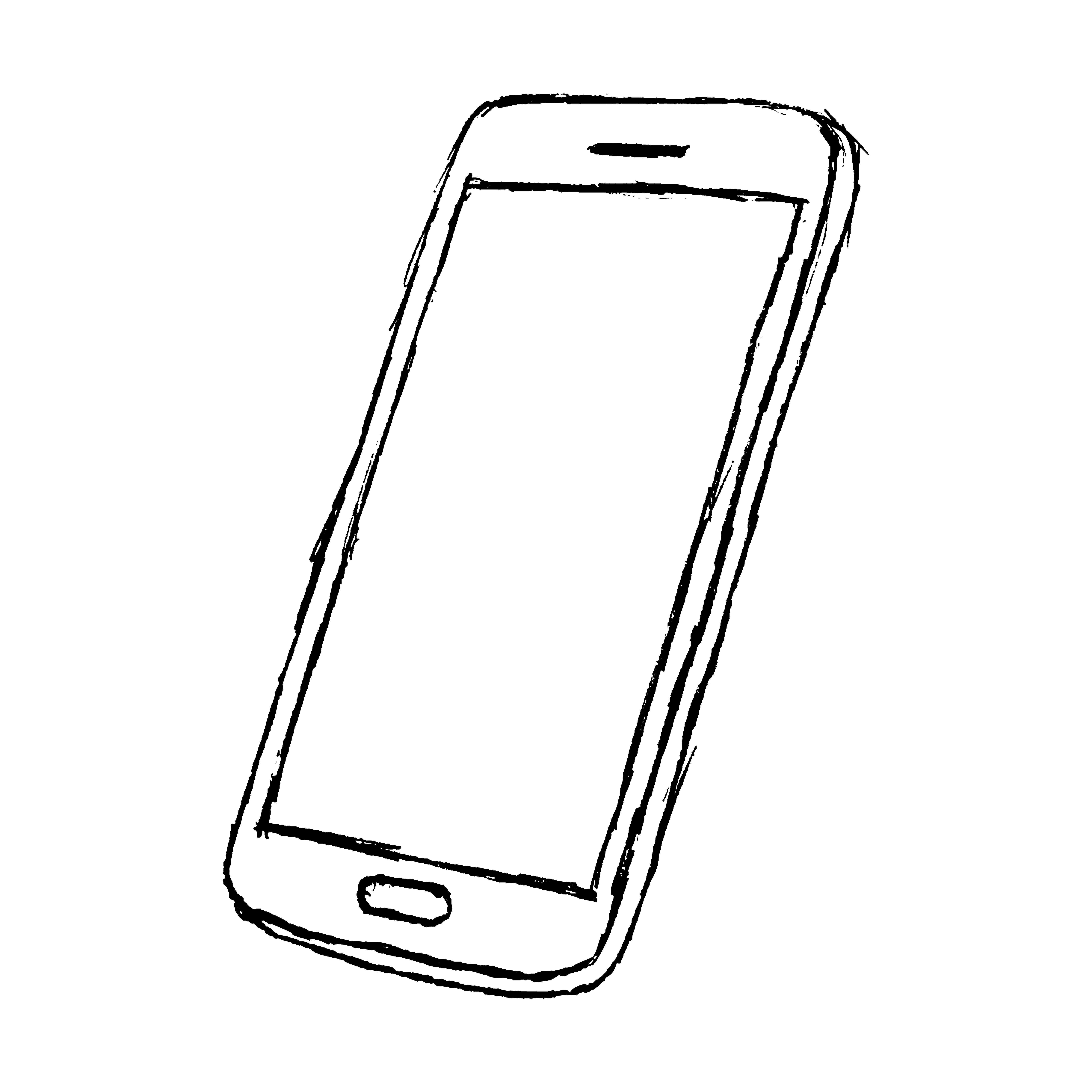The image is a black and white line art drawing of a smartphone, positioned on a clean, white background. The phone, which resembles an older model Android with some iPhone-like characteristics, has a roughly sketched appearance marked by dark, bold lines. Its body outlines are rectangular with rounded corners, giving a simplistic yet detailed representation. The screen is depicted as a central rectangle, devoid of any graphics or icons. At the bottom of the phone, there's an oval-shaped home button, and at the very top, a thicker black line indicates the speaker. The sketch's slight pixelation and scratchy texture suggest it may have been scanned or copied with adjustments to brightness and contrast, yet it retains a crisp, edited look. The drawing captures a basic, monochromatic essence of the phone with a 3D bezel effect that hints at the device's thickness.